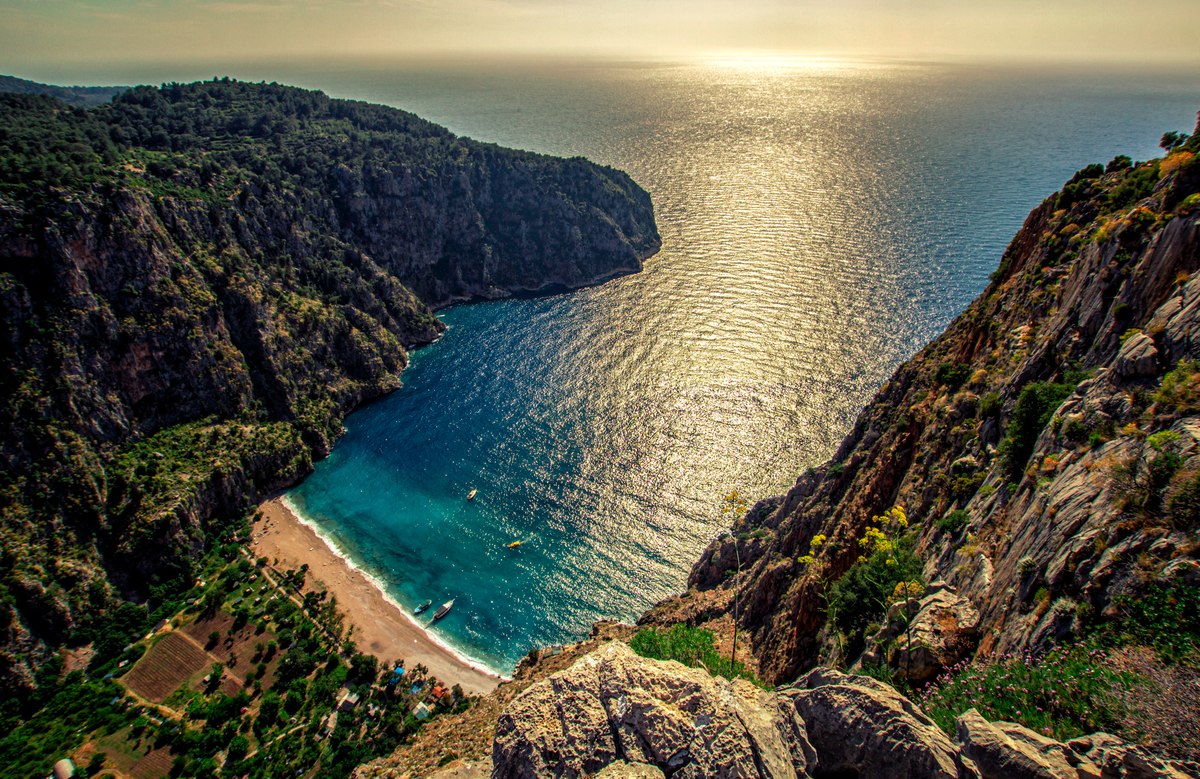This image is a vertical, rectangular shot of a picturesque bay surrounded by mountains and the ocean. At the very top, occupying the upper 10% of the image, is a sky with a soft yellow glow suggesting either sunrise or sunset, with a subtle cloud overcast. The sun is centered in this portion, casting a reflection that dances across the water below.

The bay itself is a small, rectangular area nestled between two steep, rocky mountain cliffs that extend into the ocean. These cliffs are primarily composed of dark gray rock interspersed with patches of grass and shrubs, giving them a rugged appearance. The left mountain is not as tall as the one on the right.

The water in the bay transitions from the sun's reflective glow to hues of blue and green. Below the cliffs lies a small beach with brown sand and some sparse trees scattered around. The beach seems to host a few people enjoying the scene. Several boats are anchored in the bay, and off to one side, there appears to be a small fishing village, adding a touch of human activity to this serene landscape.